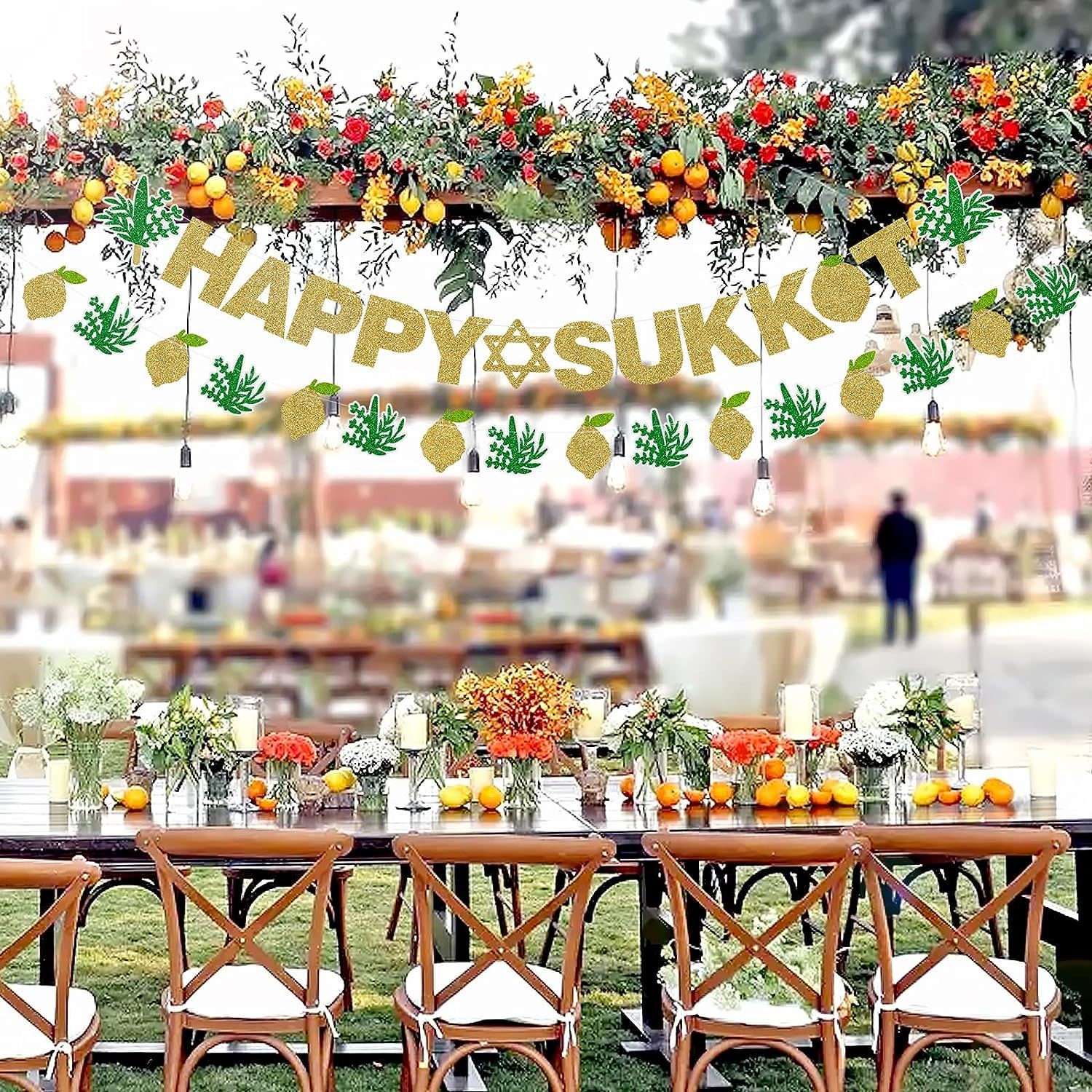The photograph captures a vibrant and festive Sukkot celebration, centered around a beautifully decorated table. Overhead, an arbor is adorned with a lush array of orange and yellow flowers, greenery, and dried oranges and lemons, creating a rich tapestry of autumn colors. A prominent banner hangs from the arbor, reading "HAPPY SUKKOT" in elegant gold letters, punctuated by a Star of David in the center. Beneath this, another decorative banner features alternating cutouts of stylized fruits and green leaves. The table below mirrors the arbor's decorations with an assortment of fresh lemons and oranges interspersed among white candles in hurricane glasses, further enhancing the festive atmosphere. Surrounding this long glass table are brown chairs with white seat cushions. The background is softly out of focus, revealing additional similarly decorated tables and a distinct figure dressed in black, contributing to the communal and joyous ambiance of the celebration.